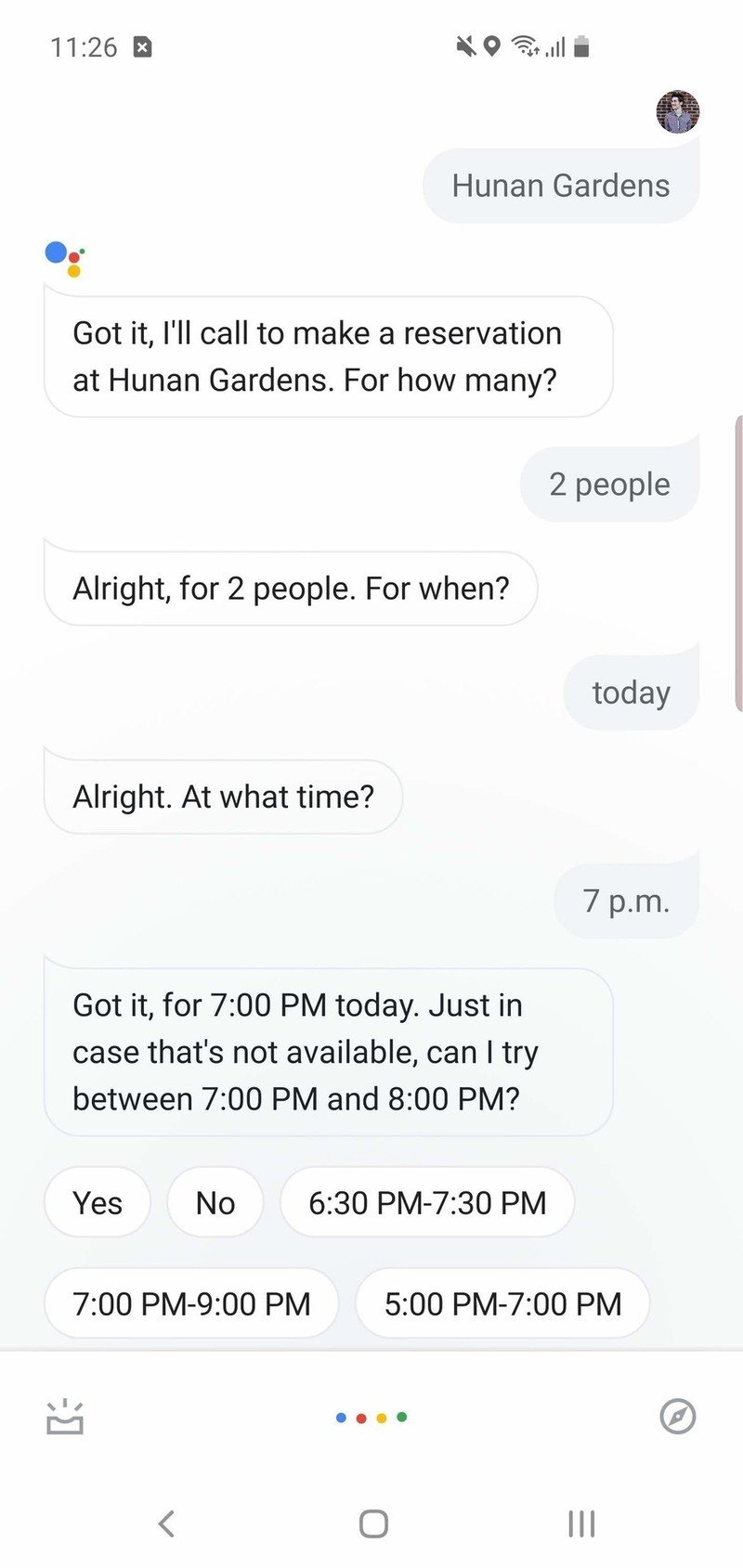**Detailed Caption:**

This image is a screenshot of a chat interface from a mobile application. The background is predominantly white, providing a clean and minimalistic look. The chat features messages from two entities, with messages from a user displayed on the right side and messages from either another person or a bot displayed on the left side.

The user messages on the right have a light gray background, while the messages on the left have a white background, maintaining a visual distinction between the two participants. At the top right corner, there is a profile picture of the user, identified as "Hunan Gardens." Opposite this, the profile picture on the left side has a white background with a circular logo containing blue, red, yellow, and green colors, typically indicative of a bot or service avatar.

The chat follows an alternating pattern, initiating with the user at Hunan Gardens:
1. "Got it, I'll call to make a reservation at Hunan Gardens."
2. From the bot: "For how many?"
3. User: "Two people."
4. Bot: "Alright, for two people, for when?"
5. User: "Today."
6. Bot: "Alright, at what time?"
7. User: "7pm."
8. Bot: "Got it, for 7pm today. Just in case that's not available, can I try between 7pm and 8pm?"

Beneath this final message, there are several response options presented to the user on white pill-shaped buttons with black text. These options are visually organized into two rows:
- The first row includes, from left to right: "Yes," "No," "6:30pm to 7:30pm."
- The second row includes: "7pm to 9pm," and "5pm to 7pm."

The footer of the chat interface is separated from the rest of the screen by a thin gray line. This section includes, on the left, a gray rectangle with a concave top and three gray lines radiating from it, symbolizing a sound or settings icon. To the right of this icon are four color-coded dots (blue, red, yellow, green) arranged horizontally. On the right side of the footer sits a gray compass icon, completing the interface's navigation tools.